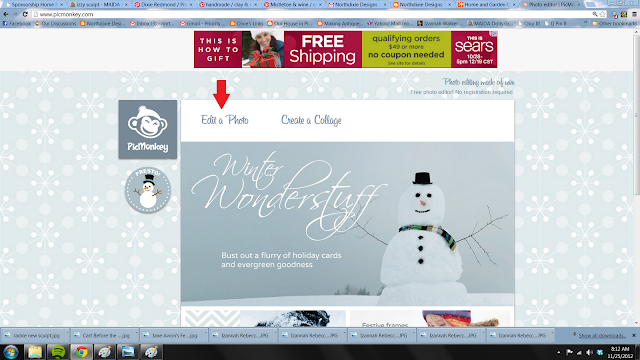In this somewhat blurry screenshot of a browser window taken on a Windows operating system, various interface elements and icons are visible. Starting from the bottom left corner, the iconic Windows logo, composed of the four colors orange, blue, green, and yellow, marks the start menu. Adjacent to this, several program icons are lined up, including older icons of Spotify, Google Chrome, Microsoft Paint, a photo app, and another paint application.

In the bottom right corner, the system clock indicates the time as 8:12 a.m. on November 25, 2012. Just above this, a "Show all downloads" prompt is visible, alongside a list showing approximately eight downloaded items. Moving to the top right of the image, the standard browser control buttons for exit, minimize, and expand are clearly seen.

The user has eight or nine browser tabs open, with the active tab displaying a webpage for "Pig Monkey." Centrally featured in the screenshot is an image of a snowman, enclosed within a square frame. This snowman is adorned with a black hat and a scarf featuring green, white, and blue stripes. It has bright, expressive eyes, a carrot nose, and twig arms. To its left, in white text, the phrase "Winter Wonder Stuff" is inscribed.